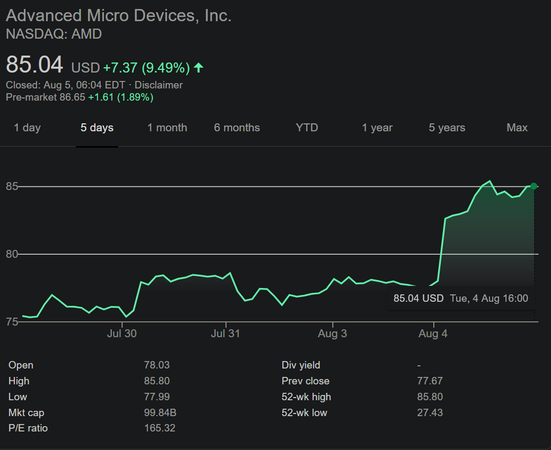The image displays the stock information for Advanced Micro Devices, Inc. (NASDAQ: AMD) against a black background. In the upper left corner, it shows the stock name and market symbol, along with the current price of $8,504 USD. The latest change is indicated in green, showing an increase of 7.37 points (9.49%) with an upward arrow. The status indicates the market is closed as of August 5 at 6:04 EDT, and the pre-market price is $86.65, also noted in green with an increase of 1.61 points (1.89%).

The upper section of the image features a line graph with options to view the stock performance over different time frames: one day, five days, one month, five months, year-to-date, one year, five years, and maximum. The five-day view is selected. The graph provides date markers at the bottom, including July 30, 31, August 3, and August 4. On August 4, the price is highlighted at $8,504 USD, with a green line trending across the graph.

The bottom section of the screen lists additional stock information, including the open, high, and low prices, market cap, and P/E ratio. To the right, there are details on the dividend yield, previous close, 52-week high, and 52-week low.